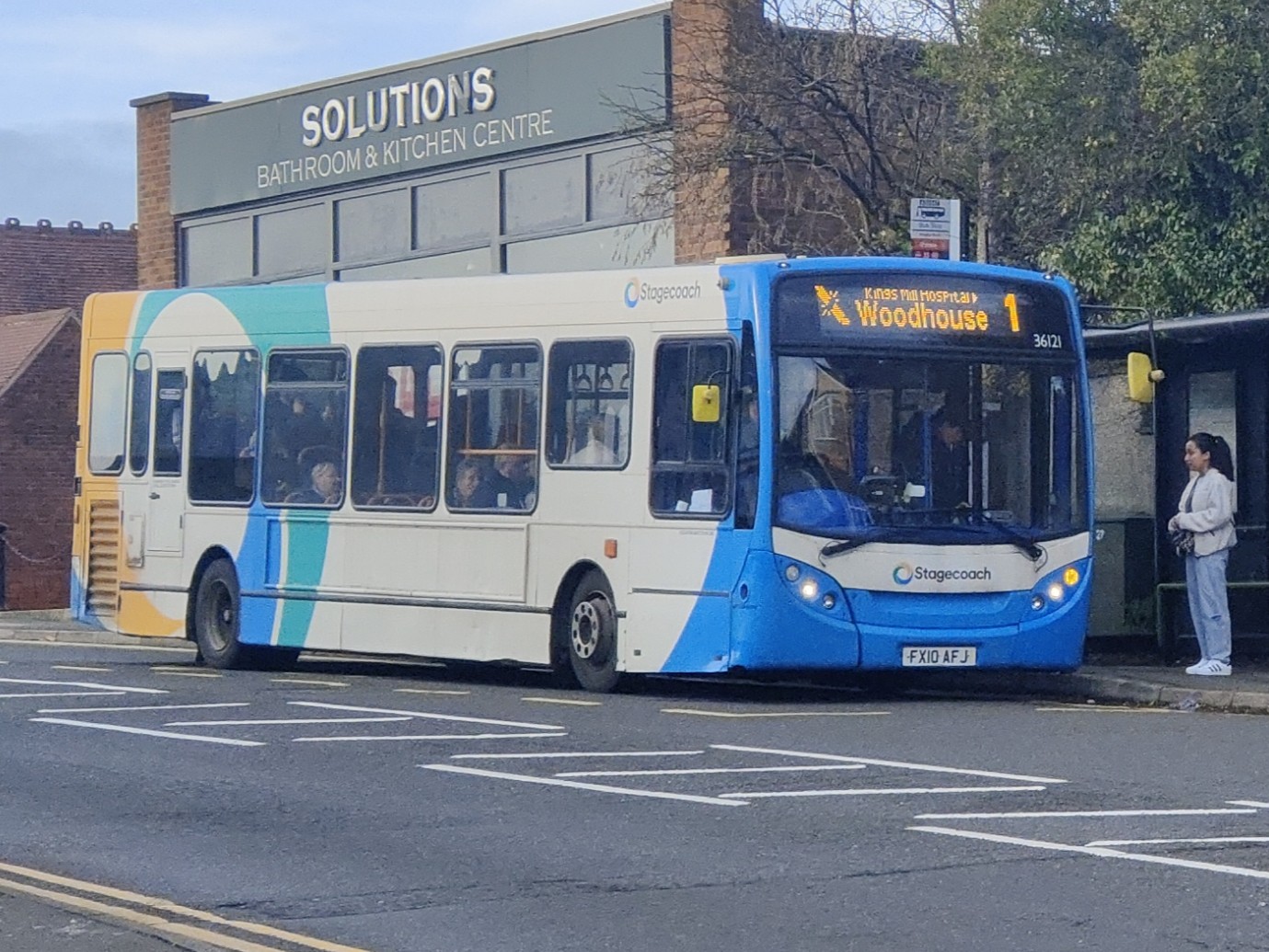In the image, a bus is prominently parked on the street in front of a building with a large sign reading "Solutions Bathroom and Kitchen Center." The bus, which features a blue front and a white rear with green, blue, and yellow swirl details, displays "Woodhouse" on its digital sign. The brand name "Stagecoach" is visible above the license plate FX10AFJ, located beneath the headlights. The bus, characterized by its flat, hoodless front and extending side mirrors, is stopped at a bus stop marked by painted white and yellow lines on the street. A woman with dark hair tied in a ponytail, dressed in a white jacket, blue jeans, and white shoes, stands on the sidewalk near the bus's front, possibly conversing with the driver through the open door. The photograph, taken on a partly cloudy day, captures this everyday urban scene in detail.